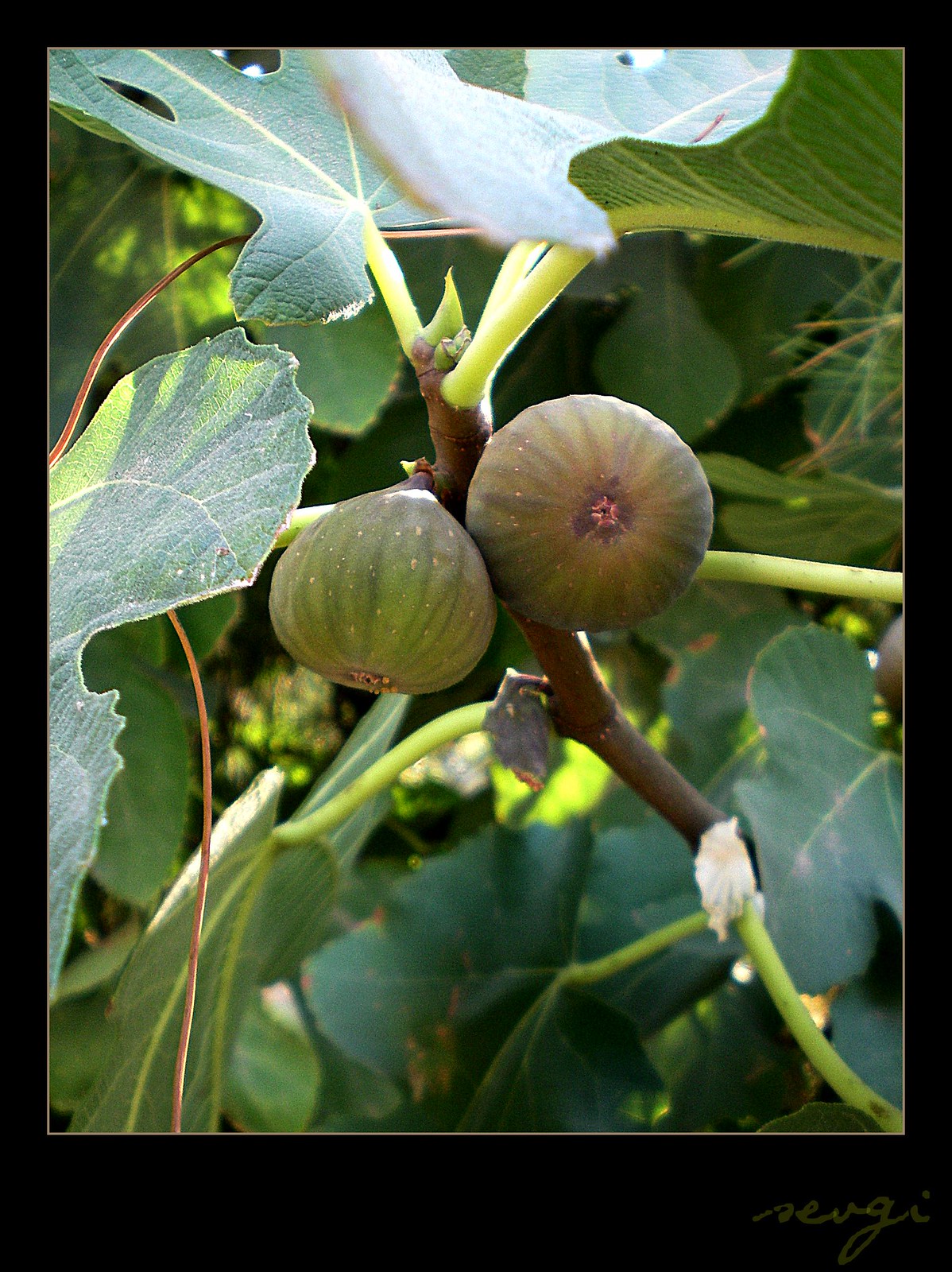This detailed photo depicts a vibrant, tropical scene. Large, dark green leaves catch the light streaming through, suggesting it was taken outdoors under bright sunlight. The primary subject is a pair of round, bulbous fruits about the size of small oranges. Though not orange, these fruits have a green-yellow hue with yellowish spots, hanging from brown, stick-like vines that emanate from the plant. In the background, light green shrubbery provides a lush backdrop, enhancing the tropical feel of the setting. Framed in a sleek black digital frame with a distinctive cursive artist's signature at the bottom, the photo captures the unique texture and coloring of the fruit and plants in meticulous detail.